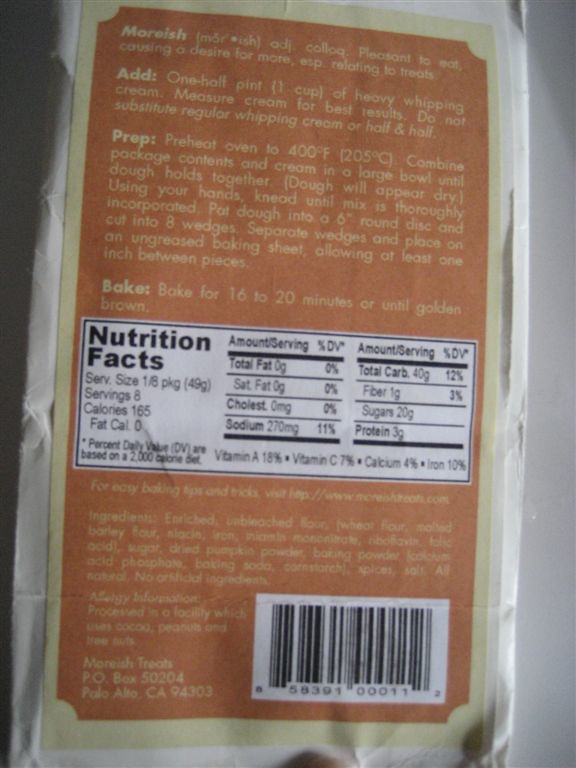The back of this food package features a vibrant label, predominantly in shades of orange-red with a touch of off-white and yellowish font for the text. At the top, the package displays the brand name "Moreish" followed by a set of detailed preparation instructions that are slightly difficult to read. 

The instructions are as follows:
1. Add 1 1⁄2 pints or 1 cup of heavy whipping cream (measure cream for best results). It specifically advises against substituting with regular whipping cream or half-and-half.
2. Preheat the oven to 400 degrees Fahrenheit (205 degrees Celsius).
3. Combine the package contents and heavy whipping cream in a large bowl until the dough begins to hold together, even though it may initially appear dry.
4. Using your hands, knead the mixture until it is thoroughly incorporated.
5. Pat the dough into a 6-inch round disc and cut into 8 wedges.
6. Separate the wedges and place them on an ungreased baking sheet, ensuring there is at least 1 inch of space between each piece.
7. Bake for 16 to 20 minutes, or until the wedges are golden brown.

Beneath these instructions, the package features a Nutrition Facts label with a white background and black font. Below the nutrition information, there is an ingredients list. The bottom of the package also contains a barcode and an address for additional information or inquiries.